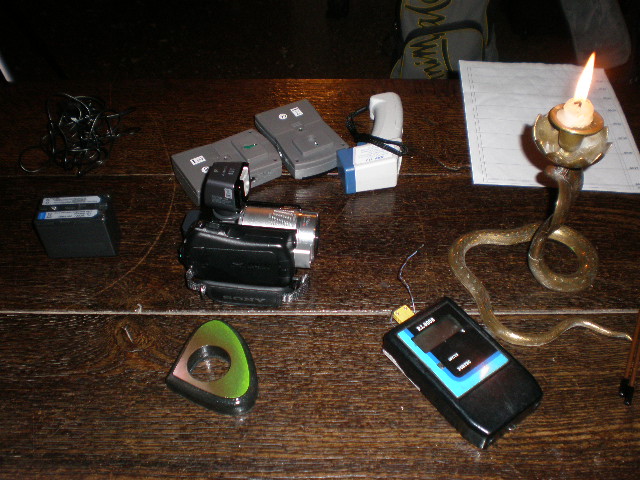This image depicts a wooden table set with an array of ghost-hunting items, suggesting an imminent paranormal investigation. Central to the composition, a nearly burnt-down white candle sits in an ornate gold or bronze candle holder shaped like a cobra, emitting a faint, eerie glow. Adjacent to the candle, a planchette rests on a Ouija board, hinting at attempts to communicate with spirits. Another intriguing artifact is a black and blue device, likely an EVP (Electronic Voice Phenomenon) recorder, used to translate ghostly energies into audible sounds. Additionally, a thermometer alongside several grey cartridges is scattered across the table, crucial tools for detecting unexplained temperature changes. A white piece of paper lies in the upper right corner of the table, potentially containing notes or instructions. The combination of these items creates an atmosphere ripe for ghost adventures, readying the space for an exploration into the supernatural.